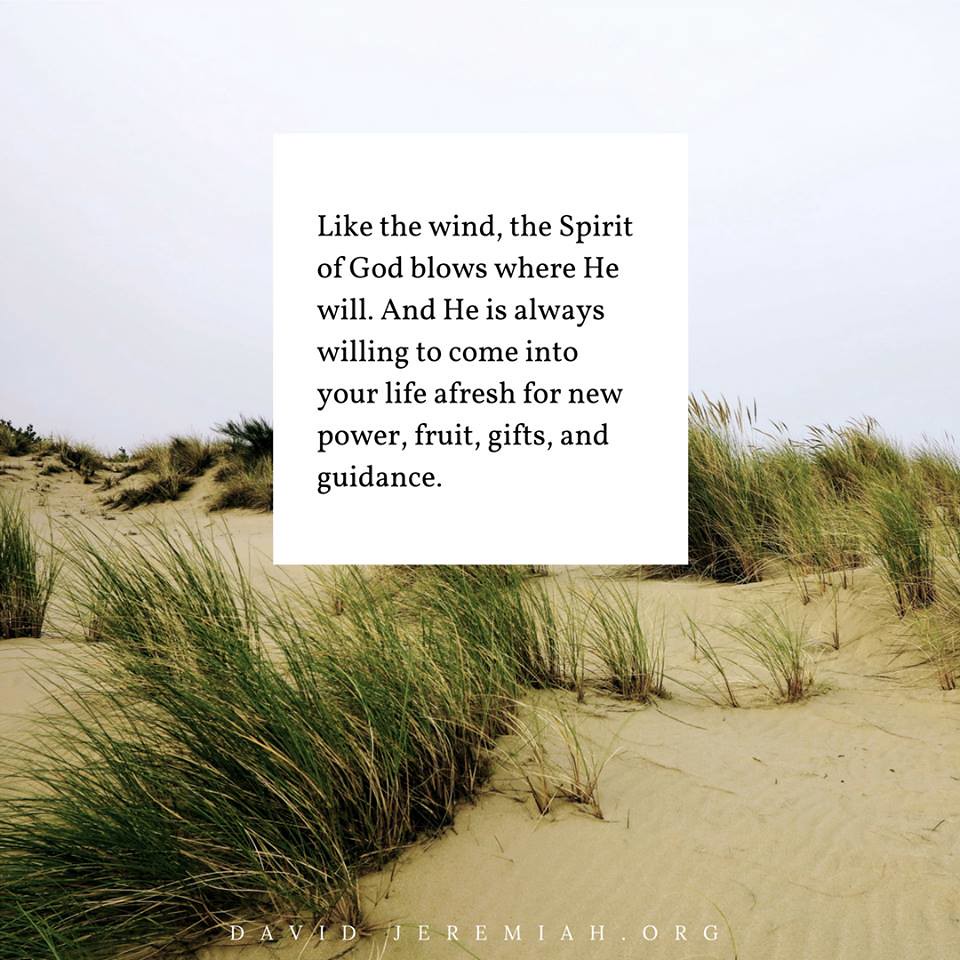This square image features a quote centered on top of a picturesque sandy scene, complete with a pale blue sky that could be entirely overcast. The sand is a light beige color, forming ripples, peaks, and valleys across the hilly dune landscape. The surface is speckled with patches of very tall, thick green grasses alongside sparse, wispy tufts and brown sticks, creating a vivid contrast amidst the sandy terrain. The grass appears to be swaying in the wind, encapsulating the essence of the quote. At the center of the image, inside a white square, the text reads, "Like the wind, the Spirit of God blows where he will. And he is always willing to come into your life afresh for new power, fruit, gifts, and guidance." At the bottom of the image, the credit “davidjeremiah.org” is clearly visible, emphasizing the source of inspiration.